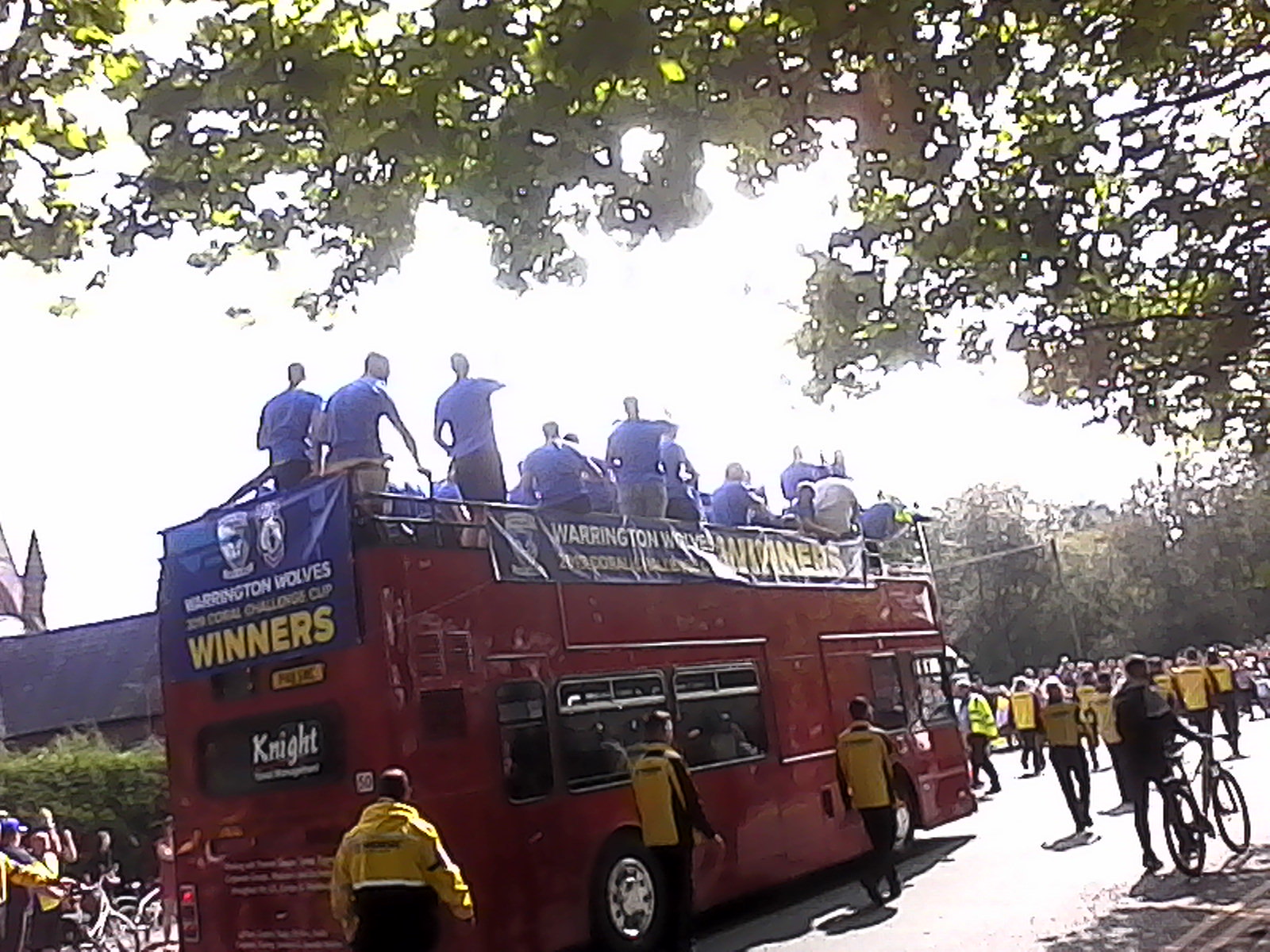This image captures a festive outdoor parade on a sunny day, featuring a striking red double-decker bus adorned with banners proclaiming "Warrington Wolves" as winners of a challenge cup, suggesting the celebrated team is a soccer squad. The bus is filled with men wearing blue uniforms, their faces obscured by backlighting from the bright sun. Surrounding the bus are individuals in yellow jackets and black pants, likely a security crew, ensuring the procession runs smoothly as it moves down the road. The scene is lively, with spectators lining the streets, some even carrying bicycles, all eagerly watching the parade. Green leaves on tree branches add a touch of natural beauty to the jubilant atmosphere.